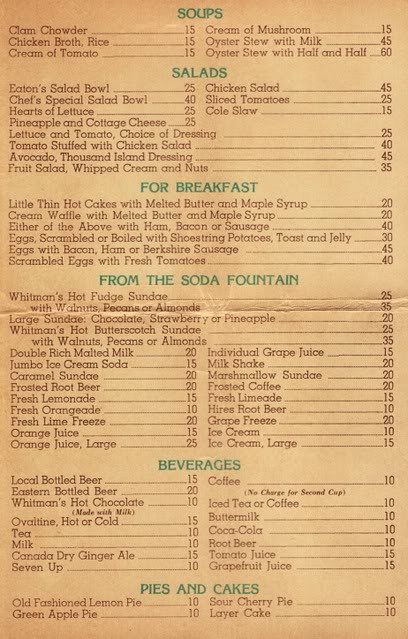The image features a vintage-style menu with a peach-colored background, displaying distinct signs of wear along a central fold mark beneath the section labeled "From the Soda Fountain." Each major category, such as "Soups," "Salads," "For Breakfast," "From the Soda Fountain," "Beverages," and "Pies and Cakes," is prominently displayed in uppercase green font, creating a nostalgic and uniform appearance. Below these headings, the specific menu items are listed in a brownish font, with the names of the dishes followed by a series of dots leading to a number, likely representing the price of each item. For example, under "Soups," offerings include clam chowder, chicken broth with rice, cream of tomato, cream of mushroom, and oyster stew available with either milk or half and half, with corresponding numbers such as 15, 15, 15, 15, 45, and 60 respectively, though the exact meaning of these numbers isn't specified. The menu design, with its straightforward presentation and traditional aesthetic, evokes a sense of dining nostalgia.